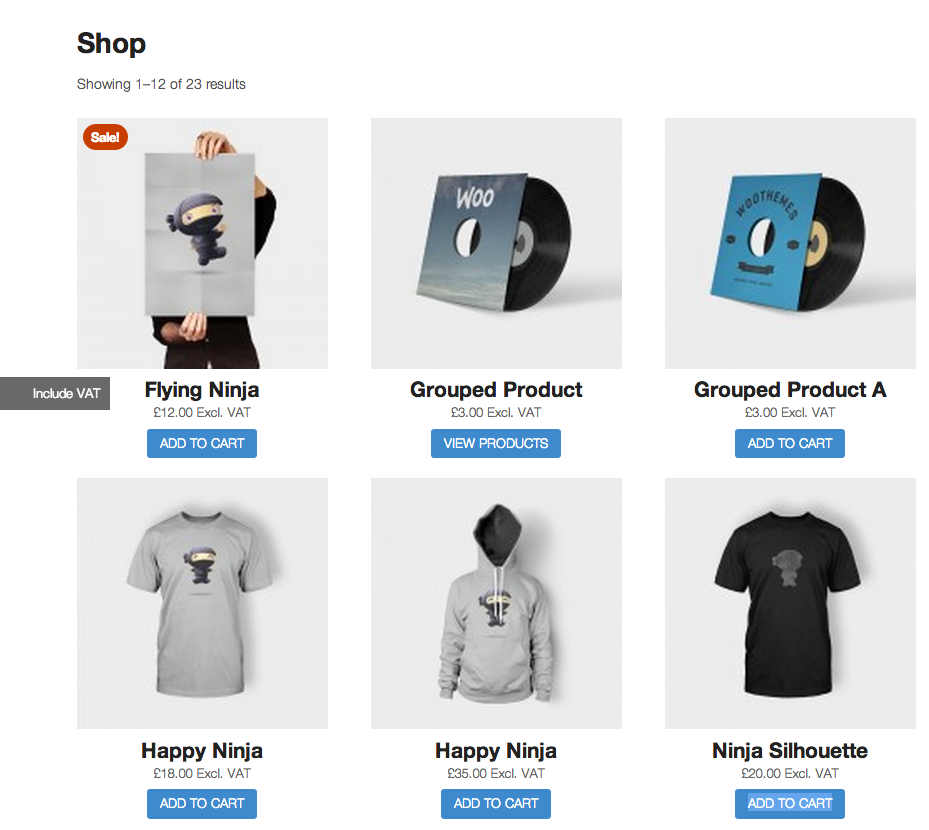The image depicts a grid layout showcasing various products available for sale online. In the top left corner, a person is holding a poster featuring a depiction of a "flying ninja." Adjacent to this, on the right, are two squares displaying musical discs, specifically vinyl records. The bottom row of the grid consists of three apparel items: a shirt on the left, a hoodie in the center, and another shirt on the right. The background features a header with the text "Shop," indicating the display of 12 out of 23 total results. On the left side, a dark blackish-gray square includes information about VAT (Value Added Tax). The majority of the products are priced in a European currency, suggesting that the store caters primarily to a European market.